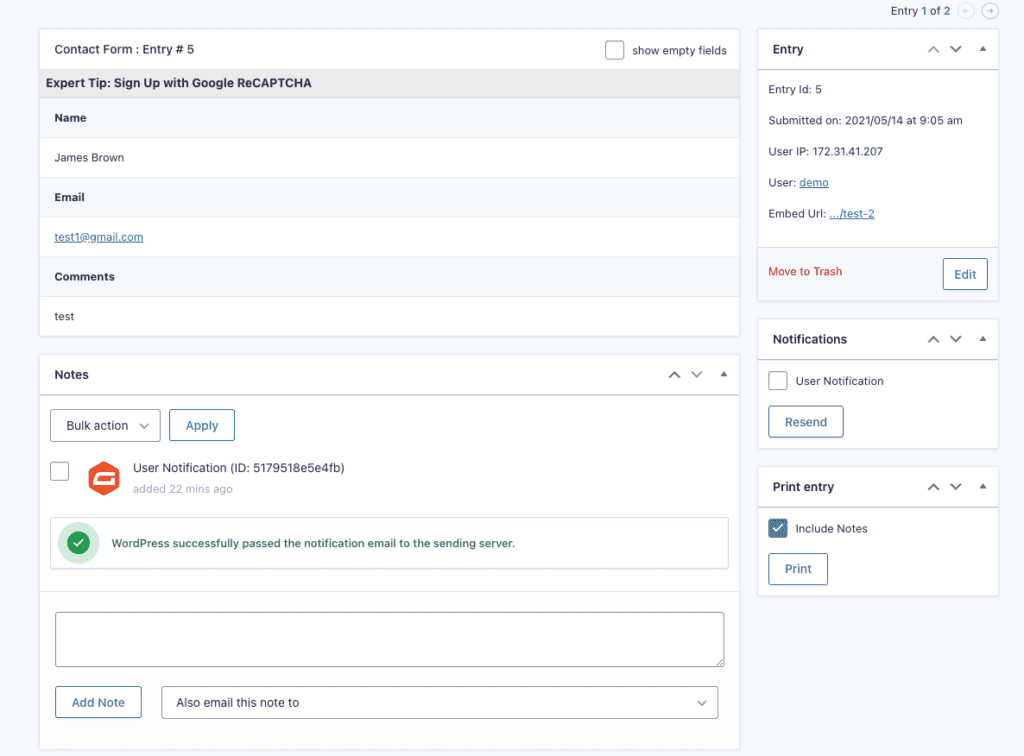This image is a screenshot from a website displaying an entry form with a focus on the submitted entry number five. 

At the top, the form begins with an area for user interaction, labeled as "Contact Form Entry Number Five." There's an expert tip suggesting users “Sign up with Google reCAPTCHA”, followed by fields for user input. The "Name" field is filled in with “James Brown,” and the "Email" field contains “test1@gmail.com”. For the "Comments" section, the word "Test" has been entered.

As one moves further down, the form includes a section labeled "Notes," which also features a "Bulk Action" dropdown menu and an "Apply" button next to it. This section is followed by an area labeled "User Notification ID" showing a long alphanumeric code indicating the unique identifier for the entry. The entry was added 22 minutes ago, as indicated by timestamp information next to an orange hexagon icon with a white letter "G" in the center, likely representing the form's integration with certain services. 

At the bottom of the form, a confirmation message states, "WordPress successfully passed the notification email to the sending server,” accompanied by a green checkmark indicating success. There are also a couple of lines available for adding a note, with a checkbox option to "Also email this note to."

On the right side of the page, details about the entry are provided: The "Entry ID" is specified as “5”, and it was submitted on May 14th, 2021, at 9:05 a.m. The right-hand side of the page continues vertically with additional details concerning the entry.